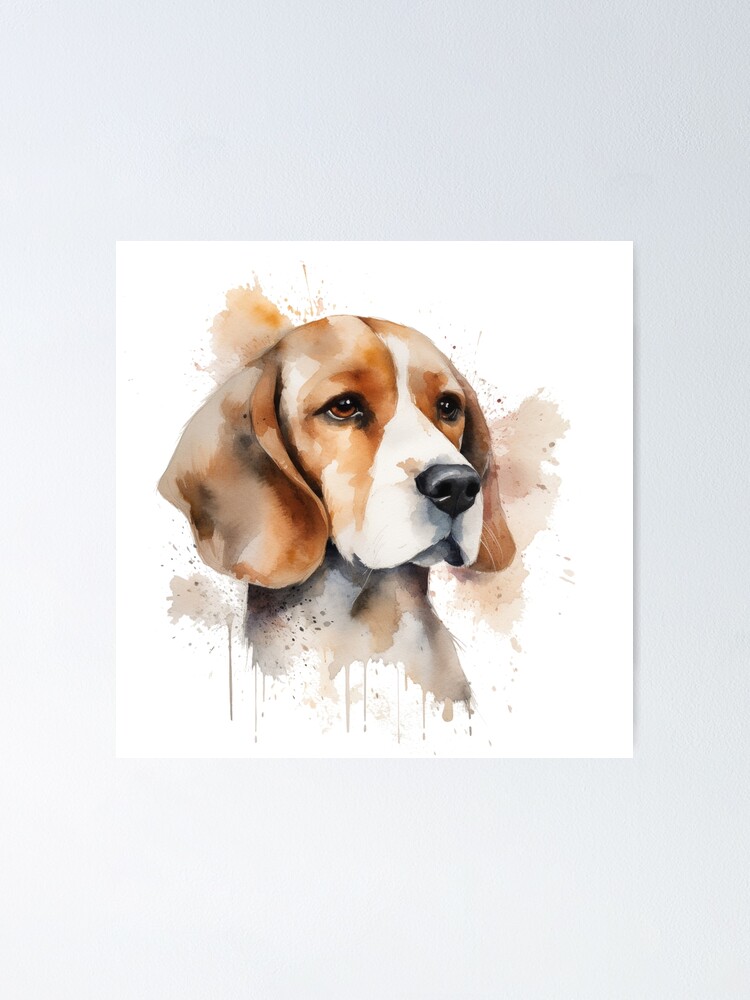This is a detailed watercolor painting of a dog, likely a hound breed such as a beagle or basset hound, displayed on a white, square canvas against a light grey wall. The dog's face dominates the composition, featuring distinctive orangish-brown ears hanging down and similarly hued fur around its eyes. A white stripe runs down the forehead, blending into a white snout accented with a black nose and noticeable dog whiskers. The attentive brown eyes are detailed with darker accents, giving the dog an expressive look. The lower part of the painting portrays the neck with shades of grey, orange, and black, transitioning into a series of artful paint splatters and drips that splatter across the bottom and right side, with a few splashes near the top left. This splattered effect lends a unique, dynamic quality to the artwork. The blending of colors and dripping paint technique give it a modern, eye-catching aesthetic, perfect for platforms like Amazon or Etsy.